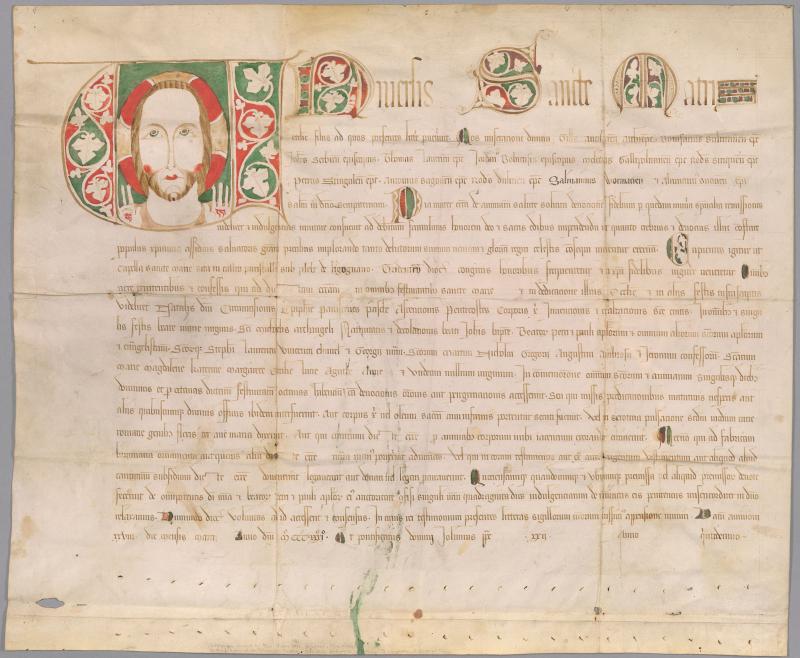This image is a color photograph in landscape orientation, depicting a page from an illuminated manuscript set against a solid gray background. The aged and worn page has a beige, tan appearance reminiscent of old parchment. In the top left corner, there is an ornate illustration featuring a long-nosed figure, likely a bearded man with brown hair, possibly portraying Christ, adorned with a red and beige headdress. His hands are raised to each side, displaying red marks on his palms. Surrounding his head are intricate red and green floral motifs, including a pattern of three leaves on either side, with a top green leaf, a red middle leaf, and a green bottom leaf. Below this illustration, the manuscript is filled with elegant, illegible Latin text written in ink, interspersed with several decorative initials throughout. The style is representational and realistic, capturing the vintage essence of the illuminated manuscript.